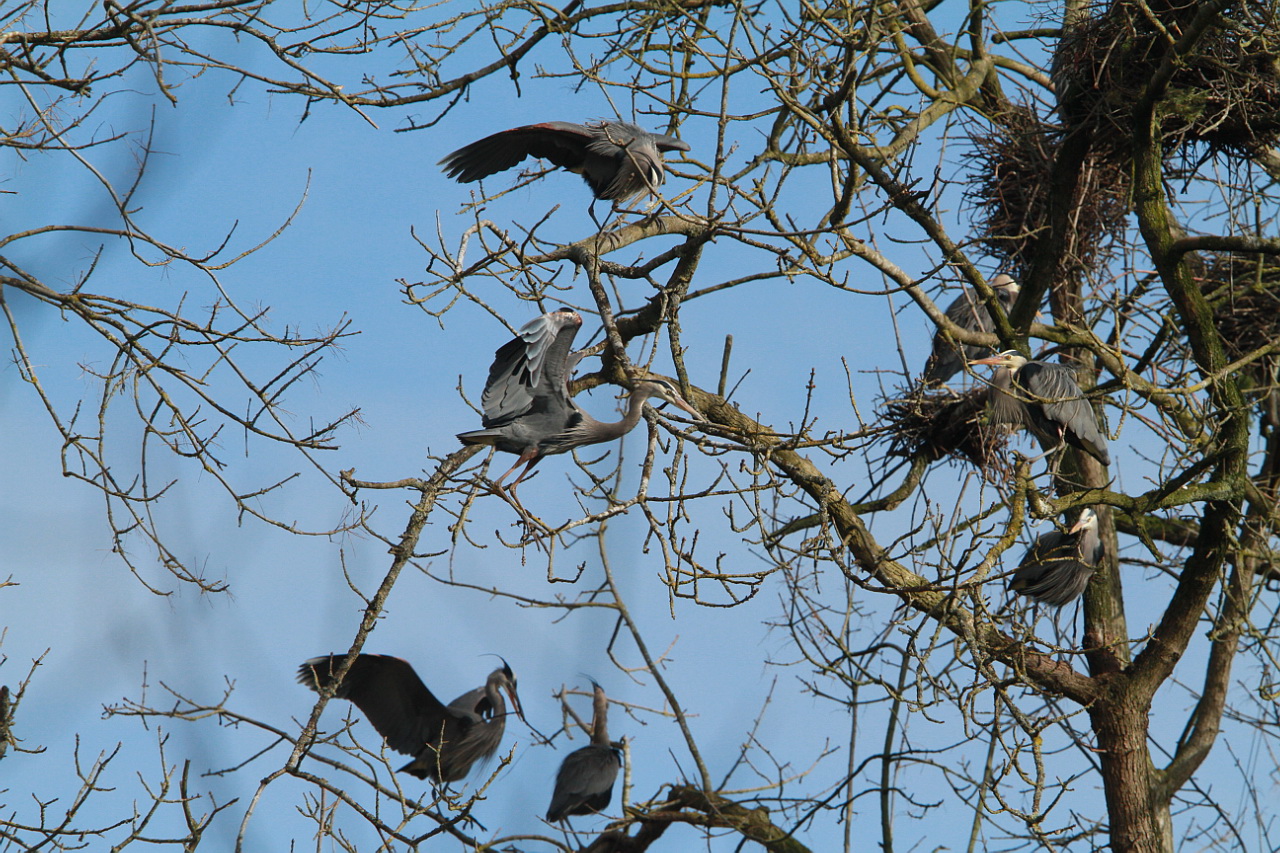In this captivating photograph, we see a dynamic scene of seven gray vultures perched and in flight, settled among the bare branches of a large tree. The tree, predominantly situated on the right-hand side with its trunk distinctly visible, stretches its slender, brown branches across the image, interspersed with some reaching in from an unseen left-side tree. At the top right of the trunk, there is a dark brown nest, suggesting a home base for these birds. The vultures, characterized by their white heads with gray streaks and striking yellow or orangey beaks, are captured in various states of roosting and motion. One vulture in the top center appears to be landing with wings outstretched, while another below looks to be taking off from its perch. Framing the scene is a serene blue sky, dotted with light gray clouds, providing a tranquil backdrop to the otherwise lively activity of the birds.